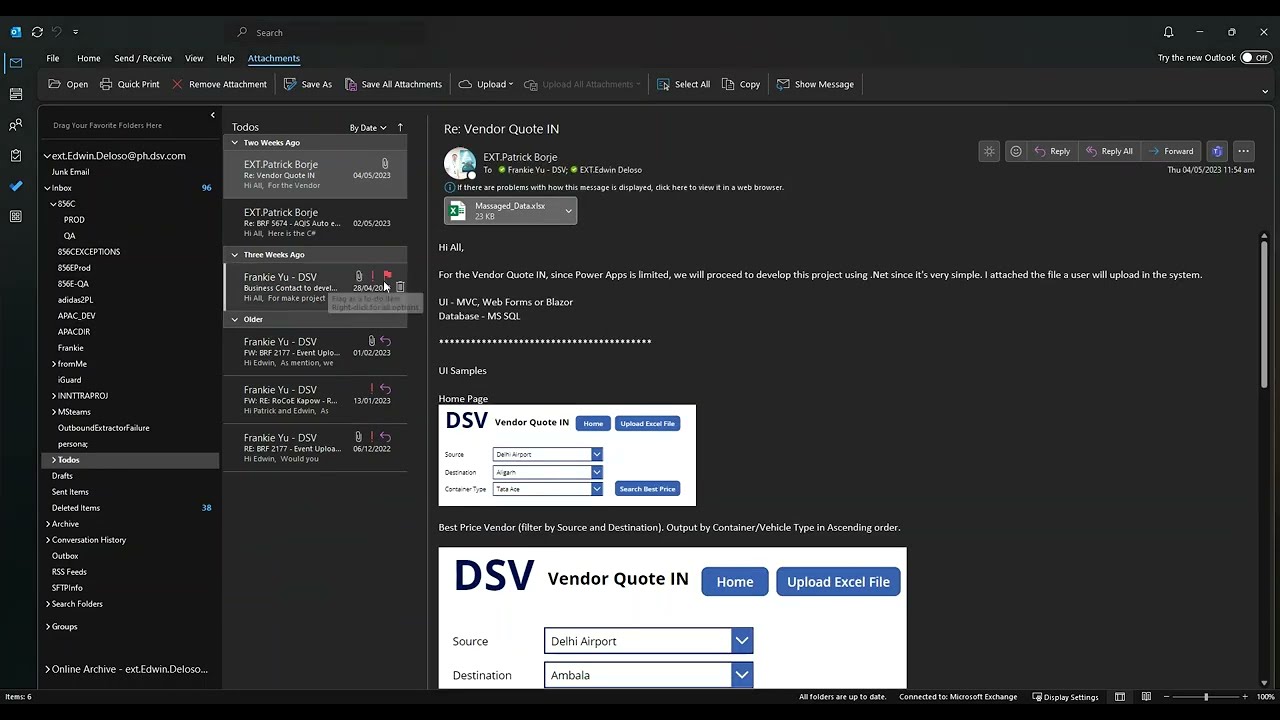This is a detailed screenshot of a computer application in dark mode, capturing someone's email interface. The toolbar at the top features categories such as File, Home, Send/Receive, View, Info, and Attachments, with Attachments highlighted in blue. On the left side, there are various folders and discussions. In the middle, an email is displayed with the subject "Vendor Quote IN," discussing the development of a product using .NET due to limitations with Power Apps. The message includes a hi all greeting and mentions an attached file. Visual elements include a white box called "DSV Vendor Quote" with blue buttons for dropdowns and options. At the bottom of the screen, typical system icons like volume control are visible.